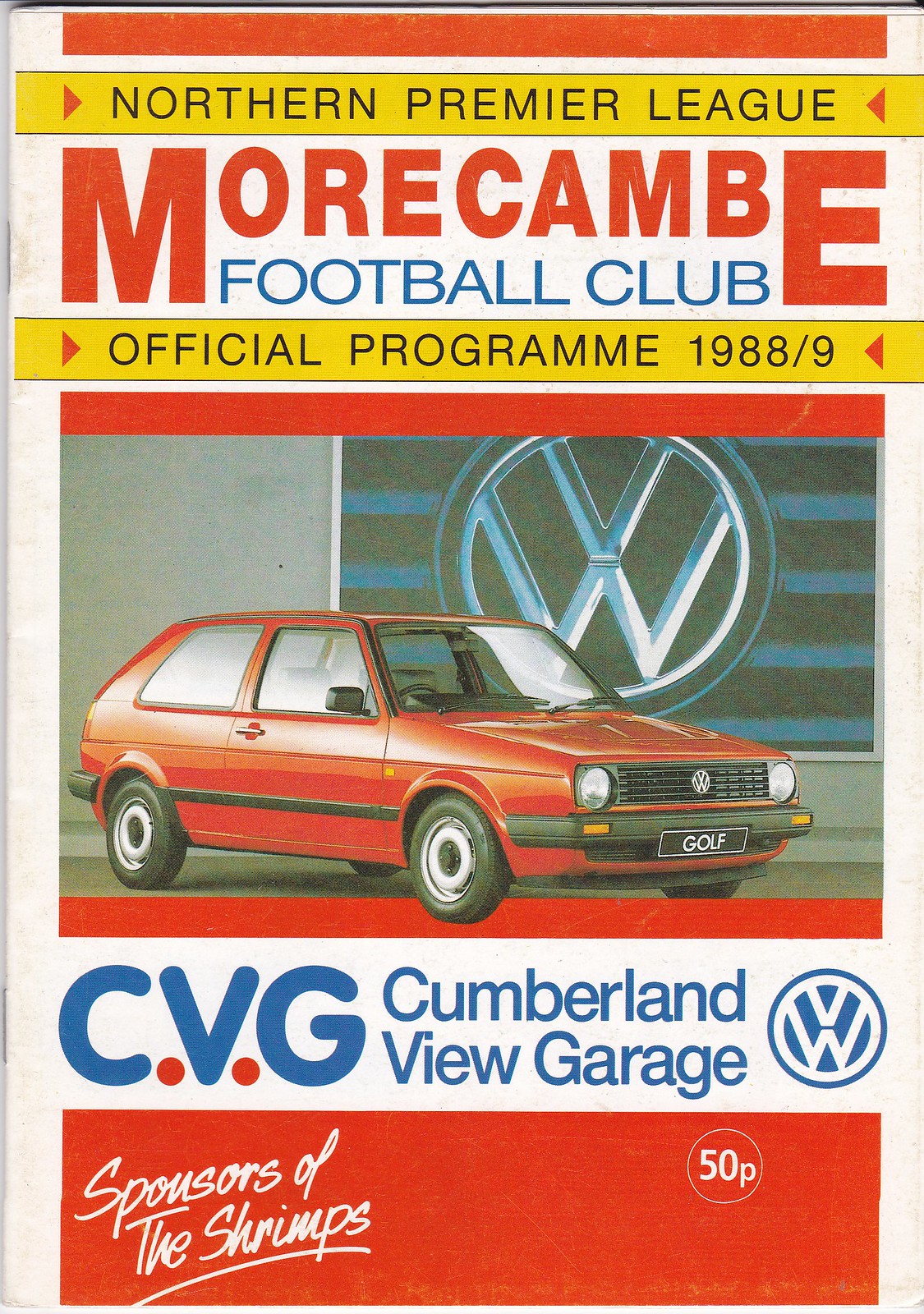The cover of this 1988-89 Northern Premier League official program prominently features a vibrant, vintage advertisement. Dominating the center is a red Volkswagen Golf with the iconic blue and white VW logo prominently displayed behind it on a flag with black and blue stripes. The top of the cover is bordered by a yellow band housing small black text that reads "Northern Premier League," followed by the title "Morecambe Football Club" in bold red and blue text. Another yellow stripe below repeats "Official Program 1988/89" in black. Below the image of the car, the text "CVG Cumberland View Garage," accompanied by another Volkswagen logo, highlights the sponsors. The bottom of the cover is capped by a prominent red box with white text proclaiming "Sponsors of the Shrimps" on the left and a small circle indicating "50P" on the right.